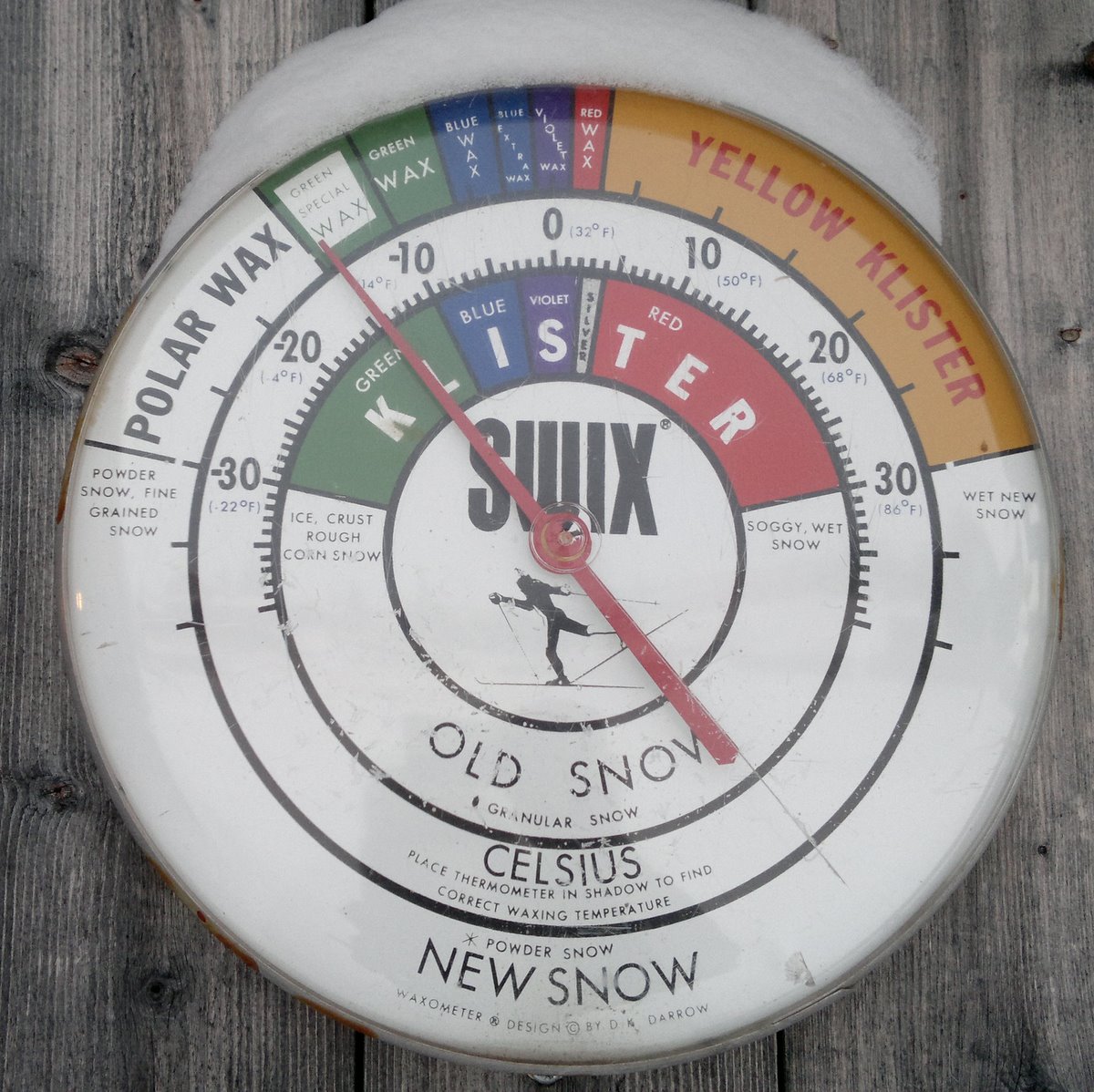This is an outdoor photograph taken during the daytime, depicting a detailed close-up of a circular weather-related meter, likely a specialized thermometer or barometer, used for assessing snow and wax conditions for skiing. The background consists of weathered gray, vertical wooden slats, with a small pile of snow resting on top of the meter.

The device is predominantly white and features a red needle pointing to the section labeled "Green Special Wax." At the very center, there's black clipart of a skier and the word "SWIX" in black letters.

Concentric circles provide various readings and information:

1. **Innermost Circle**: Displays the black skier icon and "SWIX."
   
2. **Second Circle**: Lists temperature readings from negative 30 to 30 degrees Celsius, with corresponding Fahrenheit values in parentheses beneath. The numbers are marked at regular intervals, creating individual sections for recording temperature.

3. **Third Circle**: Divided into segments by different snow conditions and associated wax types:
   - **Top Left**: "Ice Crust Rough Snow"
   - **Top Right**: "Soggy Wet Snow"
   - Colored segments for K-L-I-S-T-E-R: Green for "K-L," blue for "I," violet for "S," silver for the separator, and red for "T-E-R."
   - Labels: "Old Snow" and "Granular Snow."

4. **Outer Circle**: This ring includes various categories of snow types and waxes, specifically:
   - "Powder Snow," "Fine Grain Snow," and "Polar Wax" on the left.
   - "Green Special Wax," "Green Wax," "Blue Wax," "Extra Blue Wax" (though somewhat obscured), "Violet Wax," "Red Wax," "Yellow Klister" (with red letters), and "Wet New Snow" on the right.

Additionally, it notes practical advice at the bottom center, indicating "Celsius" and reminding users to place the thermometer in the shadow for accurate waxing temperatures. The 6 o'clock position of the outer ring reads, "Powder Snow, New Snow, Waxometer and Design, Copyright, D.B. Darrow."

Overall, this meter is both a practical instrument and a detailed display for assessing snow conditions and guiding appropriate wax selection for skiing.